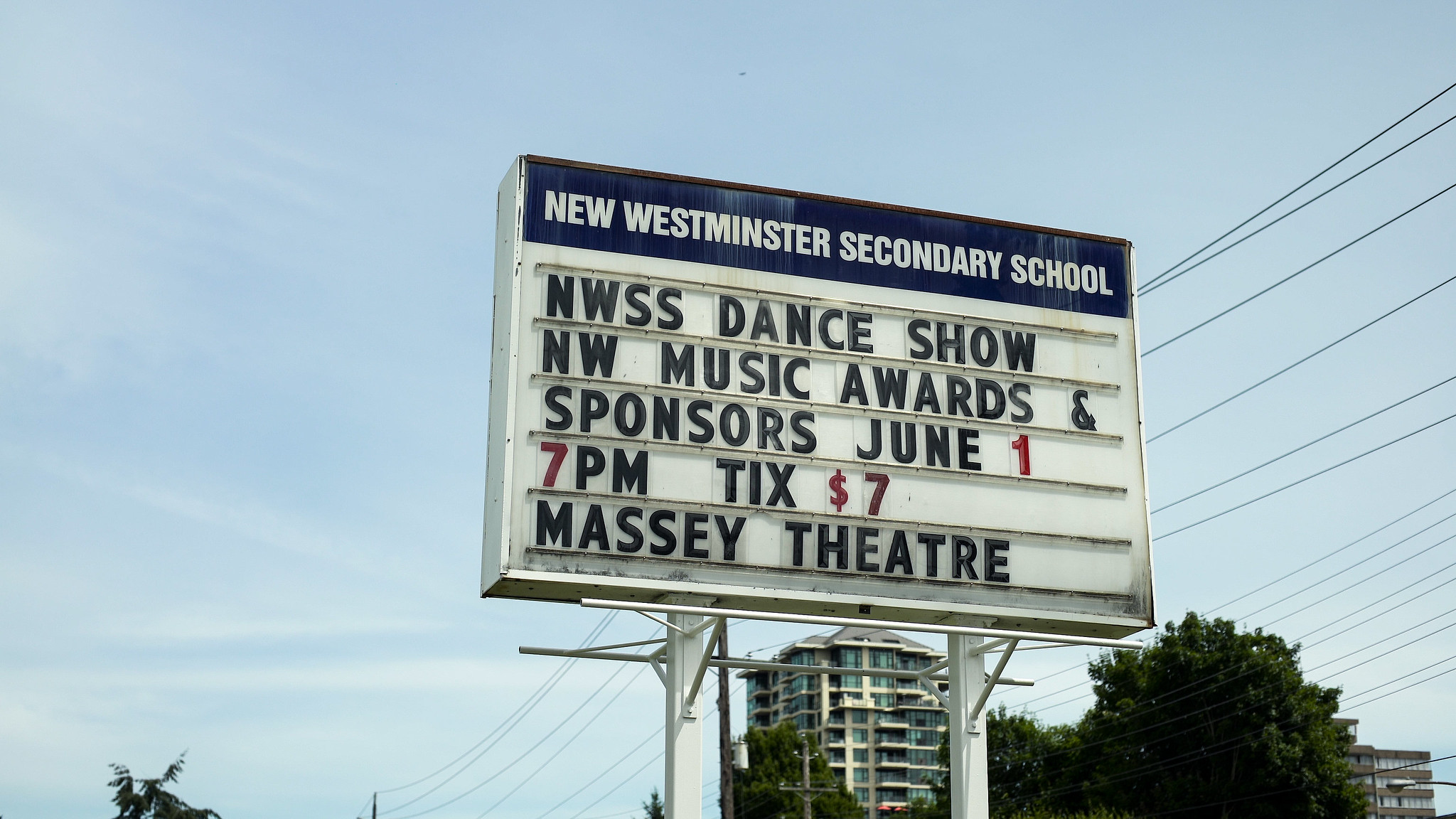This photograph captures an outdoor marquee sign for the New Westminster Secondary School, viewed from below. The sign stands on two white poles against a bright blue sky that dominates the background. Diagonally crossing the image from the bottom left to the upper right are power lines, contributing a structured element to the composition. Along the bottom of the image, more prominently on the right side, are the tops of trees and distant buildings, including plain office buildings or apartment complexes.

The sign itself has a dark blue horizontal strip at the top with white text that reads "New Westminster Secondary School." Below this, black text on a white background announces "NWSS Dance Show, NW Music Awards and Sponsors, June 1, 7 p.m., Tix $7, Massey Theatre," with the numbers in red for emphasis. The sign, showing signs of age with a slightly rusty texture, stands as a focal point amidst an otherwise clear and expansive sky, punctuated only by a few clouds.